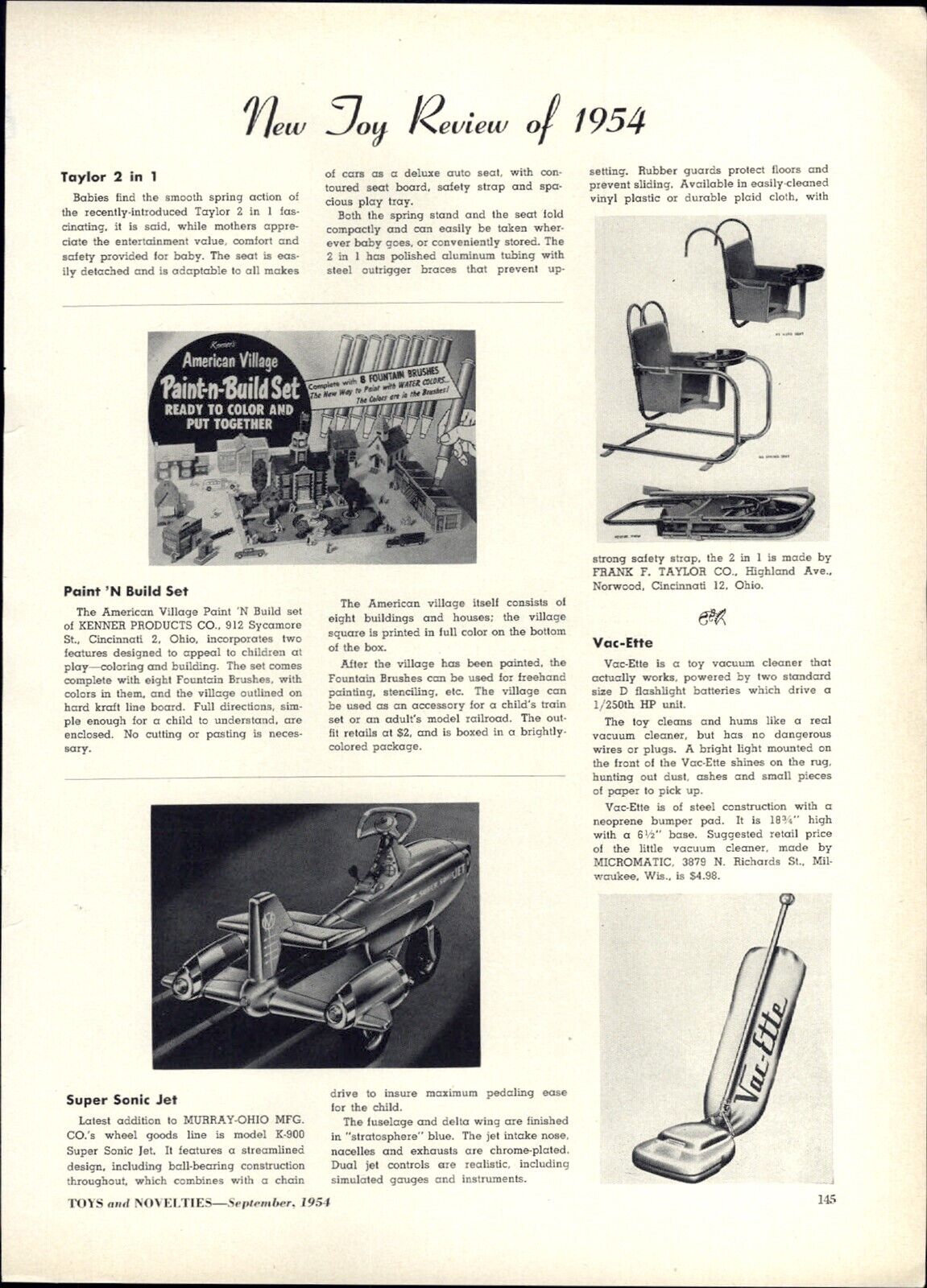The image depicts a vintage black and white magazine article titled "New Joy Review of 1954." The page shows signs of aging, with the paper darkened to a pale brown, off-white hue. Prominently featured is the Taylor 2-in-1, a toy described as having a smooth spring action suitable for babies. Below this, a "Paint and Build Set" is displayed, marketed under the name "American Village," ideal for children to color and assemble model houses. To the right of the article, three folding chairs are arranged, two are open and one folded at the bottom, suggesting a portable and versatile design. At the bottom left, there's an illustration of a "Supersonic Jet," a sleek pedal car with a steering wheel and knobs, appealing to young kids with its spaceship-like appearance. Additionally, the bottom right corner features the "Vacette," an upright electric vacuum cleaner with a large bag on the handle, typical of its time.